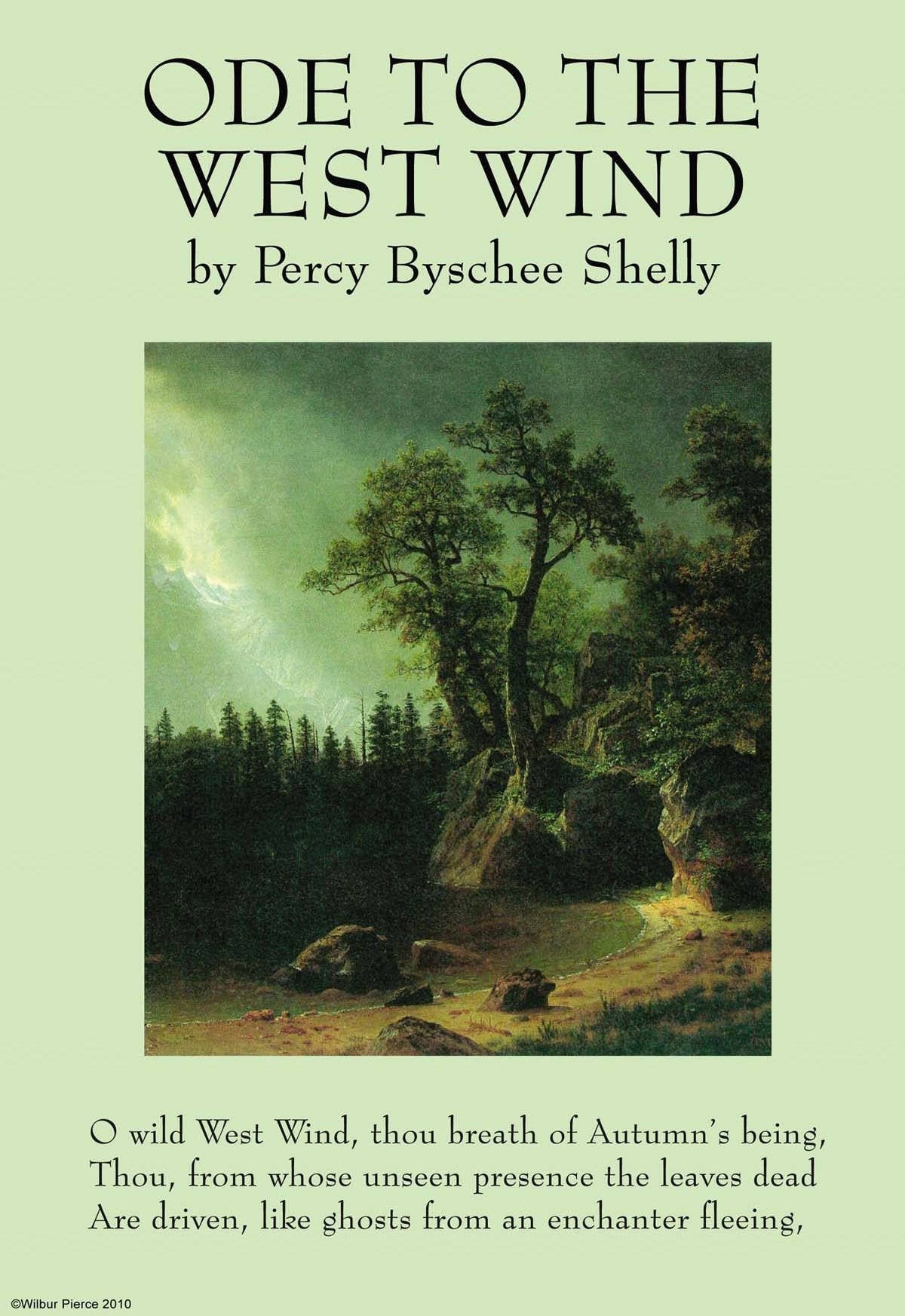This is a color photo of a book cover with a light green (pistachio) background. At the top, in bold black capital letters, it reads "ODE TO THE WEST WIND" by Percy Bysshe Shelley. Below this title is a rectangular image depicting an outdoor scene. The image, with a gray blue overcast sky, shows a dense forest of tall, dark green pine and evergreen trees, scattered rocks and stones, and a dirt path winding through a hilly area. The sky hints at a clearing with sunbeams piercing through, adding a mysterious and somber tone to the forest landscape. At the bottom of the cover, in black font, there's a poetic excerpt: "O wild west wind, thou breath of autumn's being, thou from whose unseen presence the leaves dead are driven, like ghosts from an enchanter fleeing." Additionally, in the bottom left corner of the cover, a small watermark indicates "© Wilbur Pierce, 2010."